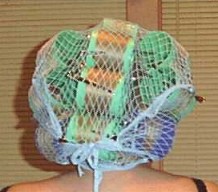This is a photograph taken from behind of a woman with blonde or light brown hair, styled in old-fashioned, light and dark green plastic curlers, alongside some blue rollers near the nape of her neck. The curlers are held in place with clips and secured under a light blue, stretchy hairnet. The woman is wearing a spaghetti strap top and a black bra strap is visible on her shoulders. The setting includes a brown wall and two windows with blinds, and there appears to be the arm of a pair of glasses on the right-hand side, suggesting she might wear glasses.